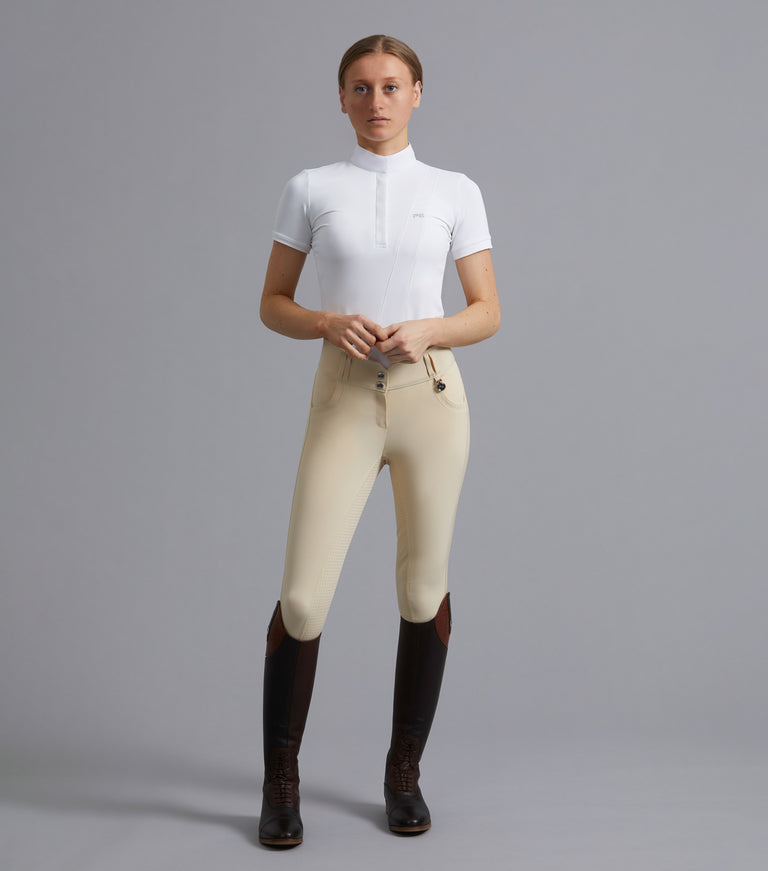The image portrays a slender, attractive Caucasian woman standing against a gray background, modeling an equestrian riding outfit. She has slicked-back, brown hair parted in the middle and blue eyes, with a serene, expressionless face. She is dressed in a short-sleeve, collared white shirt that is tucked into tight, light khaki pants, showcasing her form-fitting attire. Completing the ensemble are her shiny, knee-high brown and black boots. Her hands are resting at her sides, with fingers interlinked near her waist, emphasizing her poised and composed demeanor. The photo captures the elegance and unique style associated with equestrian sports.